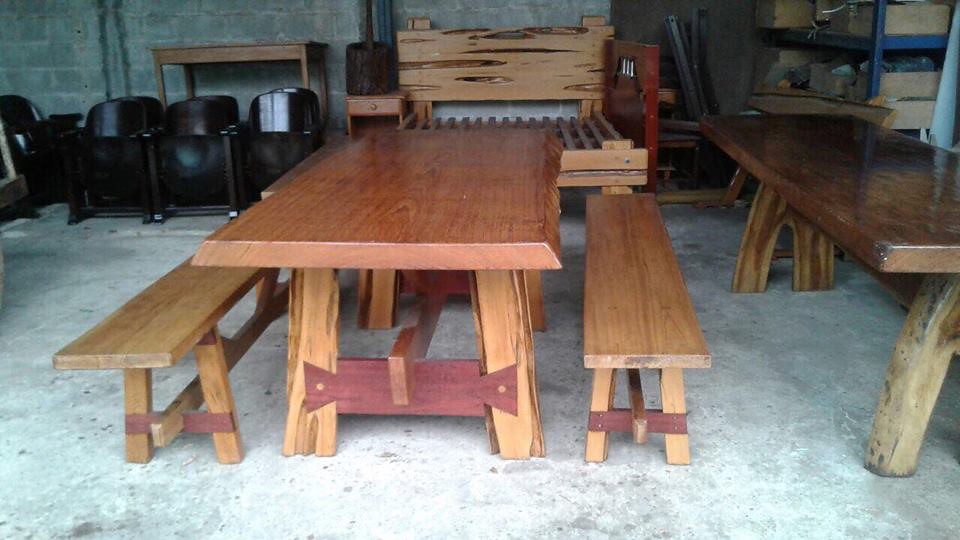The photograph portrays an indoor space that appears to be a furniture workshop or storage area with a concrete floor and walls. In the upper left corner, there is a stack of folded black chairs, reminiscent of theater seats, leaning against the wall. Nearby, shelves and boxes are visible, contributing to the cluttered ambiance of the space.

Central to the image is a large, prominently featured wooden table accompanied by a pair of matching benches on each side. The table and benches share a cohesive design, featuring a distinctive red wooden base that binds the leg areas. The furniture is substantial and robust, with the table displaying a reddish hue, while the benches exhibit a more golden tone.

To the right of this central table is another wooden table, characterized by a darker, rustic look with tree trunk-like legs, possibly indicating it is either older or crafted from natural wood with visible knots. This table contrasts slightly with the main focal piece but fits the overall wooden aesthetic of the workshop.

In the background, additional wooden furniture pieces can be seen, including what appears to be a bed frame and possibly a drawer or side table, adding to the impression that this space is dedicated to the crafting or storage of wooden furniture. The floor beneath these items is a speckled white cement, reinforcing the utilitarian nature of the space. Overall, the scene captures the essence of a busy workshop filled with various wooden furniture pieces, emphasizing the large table and benches at its core.